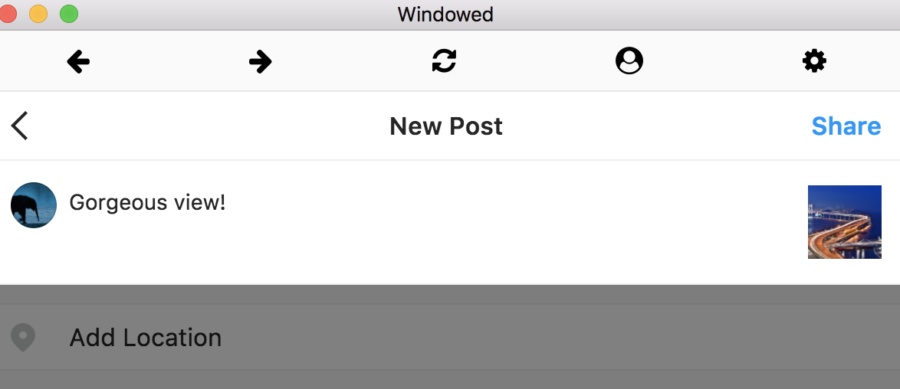Here is a detailed and cleaned-up caption for the image:

---

The screenshot appears to capture a segment of a user interface, likely from a website. At the top, there is a gray toolbar featuring three multicolored dots on the upper left corner—red, orange, and green. In the center of this gray bar, the word "Windowed" is displayed in black font. Directly below this, a white bar contains navigation and utility icons: a black left-arrow on the left, a black right-arrow to its right, followed by a refresh icon, a black circle with a white human silhouette, and a black gear icon.

Further down, there is a white rectangle with the text "New Post" written in black font. To its left is a left-pointing arrow, and to its right, the word "Share" is written in blue font. 

Beneath this, another white rectangle presents an interface element: on the left side, a small blue circle contains a silhouette of an elephant. To the right of this icon, the text "Gorgeous view!" is written in black font, and on the far right, a square thumbnail depicts an overpass on a highway at night.